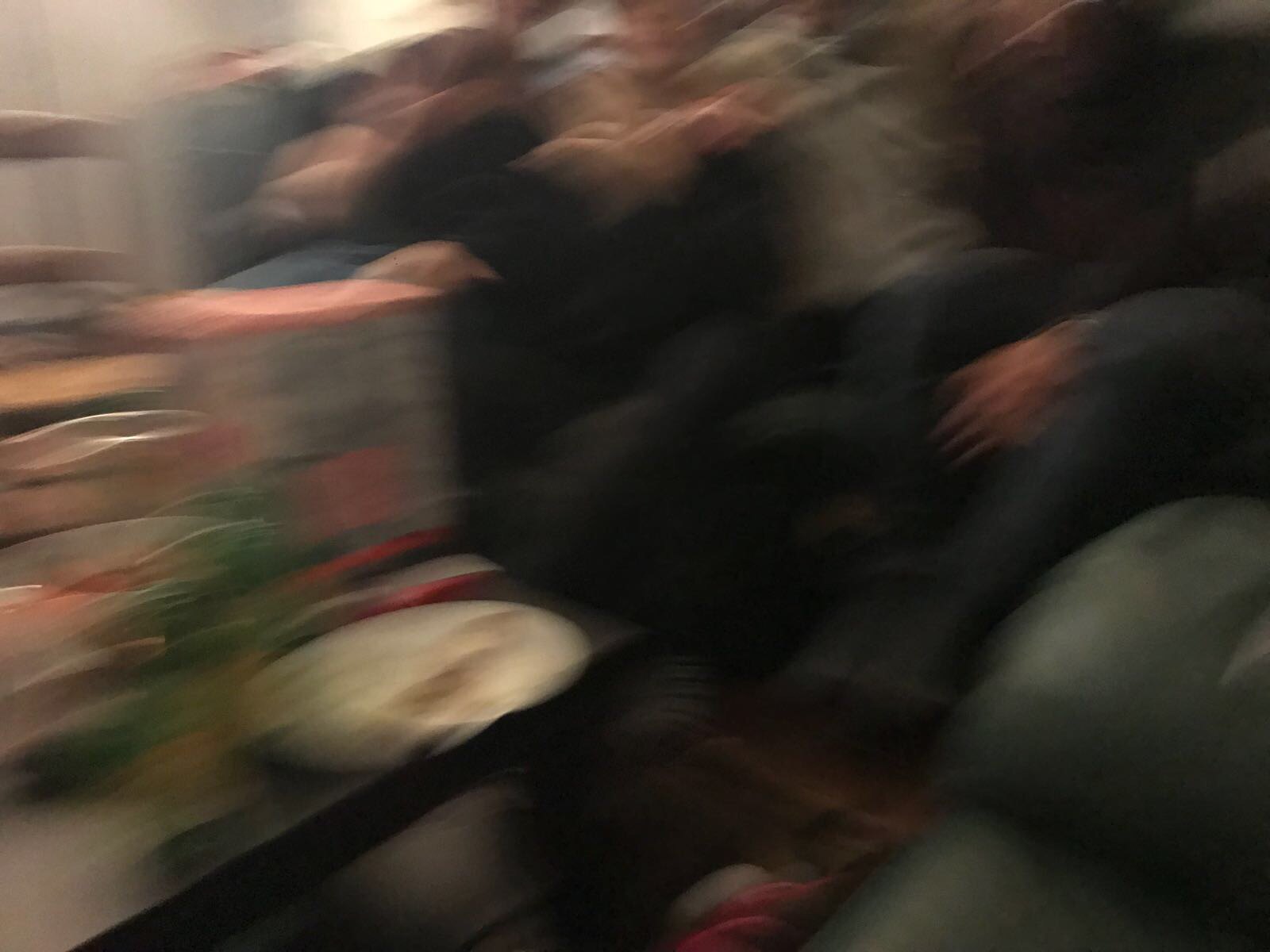In a dimly lit, cozy room, a blurry photograph captures a group of people seated across a variety of furniture pieces, their details obscured by motion blur. Central to the scene is a dark greenish sofa crowded with three or four individuals dressed in dark clothing, likely denim, their pale complexions just visible in the hazy image. In front of them, a dark brown wooden coffee table holds a white plate among other indistinguishable items, all shrouded in blur. To the left, the faint outline of a brown kitchen-style chair with distinctive crossbars can be seen. The upper left corner of the image hints at a light source, casting a dull glow over the scene, adding to the indistinct, dreamlike quality of the photograph.